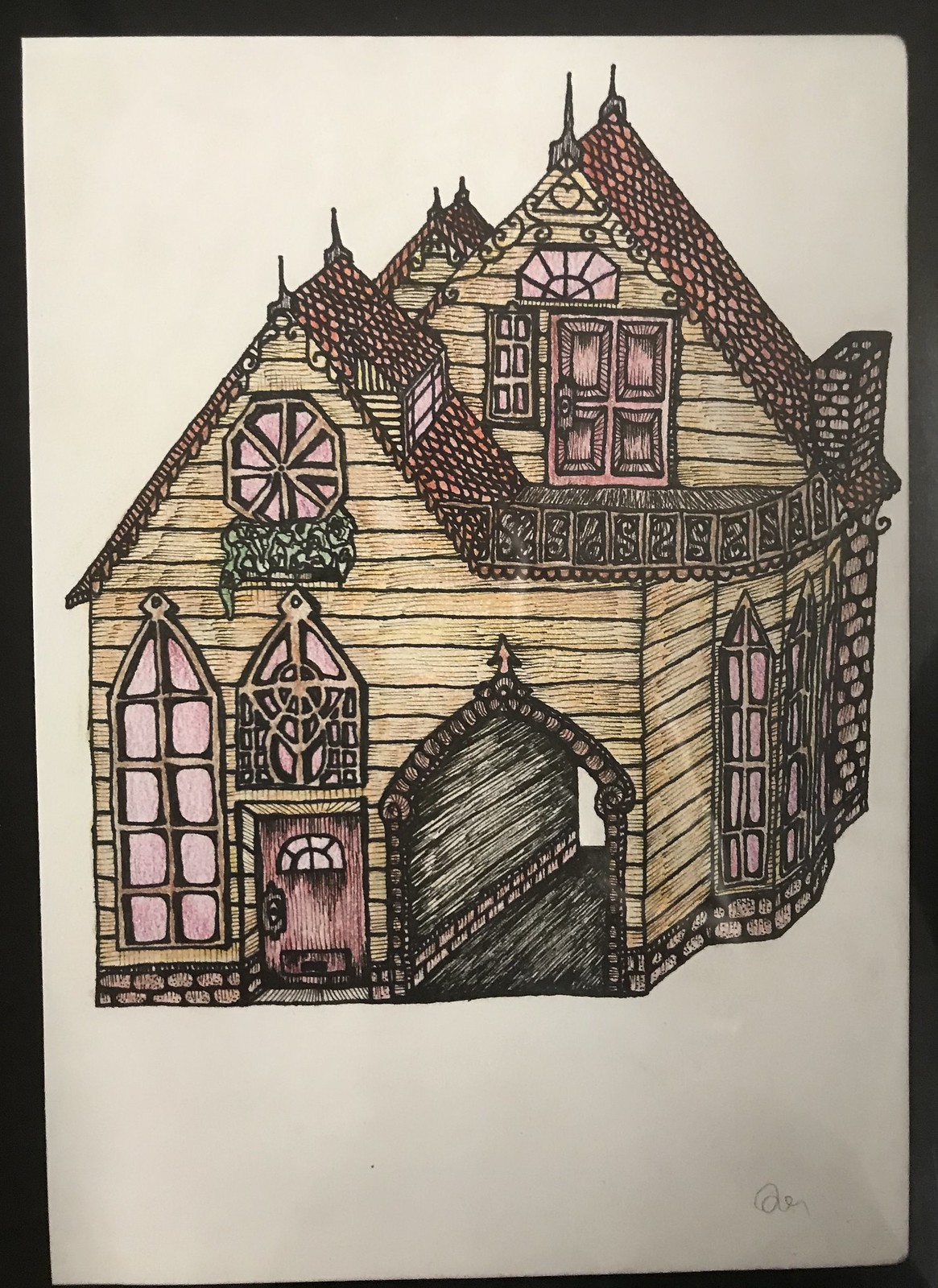This detailed drawing, sketched on white paper and slightly tilted to the left, reveals part of the black-bordered table it rests on. The illustration prominently features an A-frame house with a distinctive architectural layout. The house includes a front dormer and a central porch located on the second floor. The porch sits above an open, roofed-in driveway that leads into the house structure. The front door of the house is positioned towards the left side of the building. The sketch captures intricate details, presenting a realistic and inviting depiction of the unique home design.